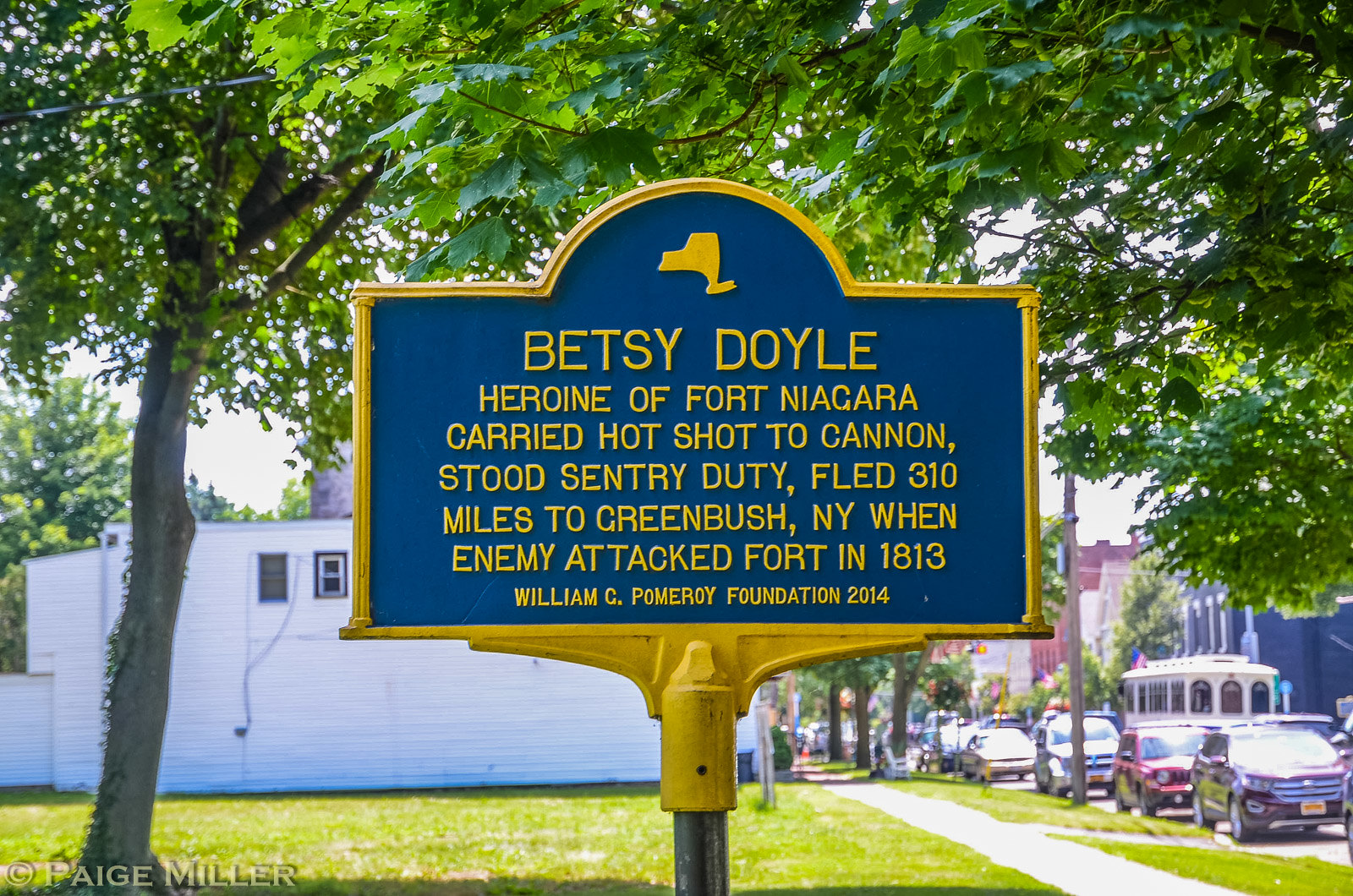This photograph captures a commemorative blue sign with a yellow outline dedicated to Betsy Doyle, heroine of Fort Niagara. The text on the sign highlights her brave actions during the 1813 attack on the fort, where she carried hot shot to a cannon, stood sentry duty, and fled 310 miles to Greenbush, New York. A symbol of New York State is located at the top of the sign, which is sponsored by the William C. Pomeroy Foundation, 2014. The sign stands on a lawn in a residential or suburban area, suggesting a neighborhood setting. Behind the sign, a large green tree, a white building, and well-manicured grass are visible, indicating a sunny day with clear, blue skies. To the right, various cars and a tour bus line the side of a street, enhancing the vibrancy of the scene. The setting appears well-maintained, featuring young trees with green foliage and a mix of older buildings in the background, lending a historic charm to the location.